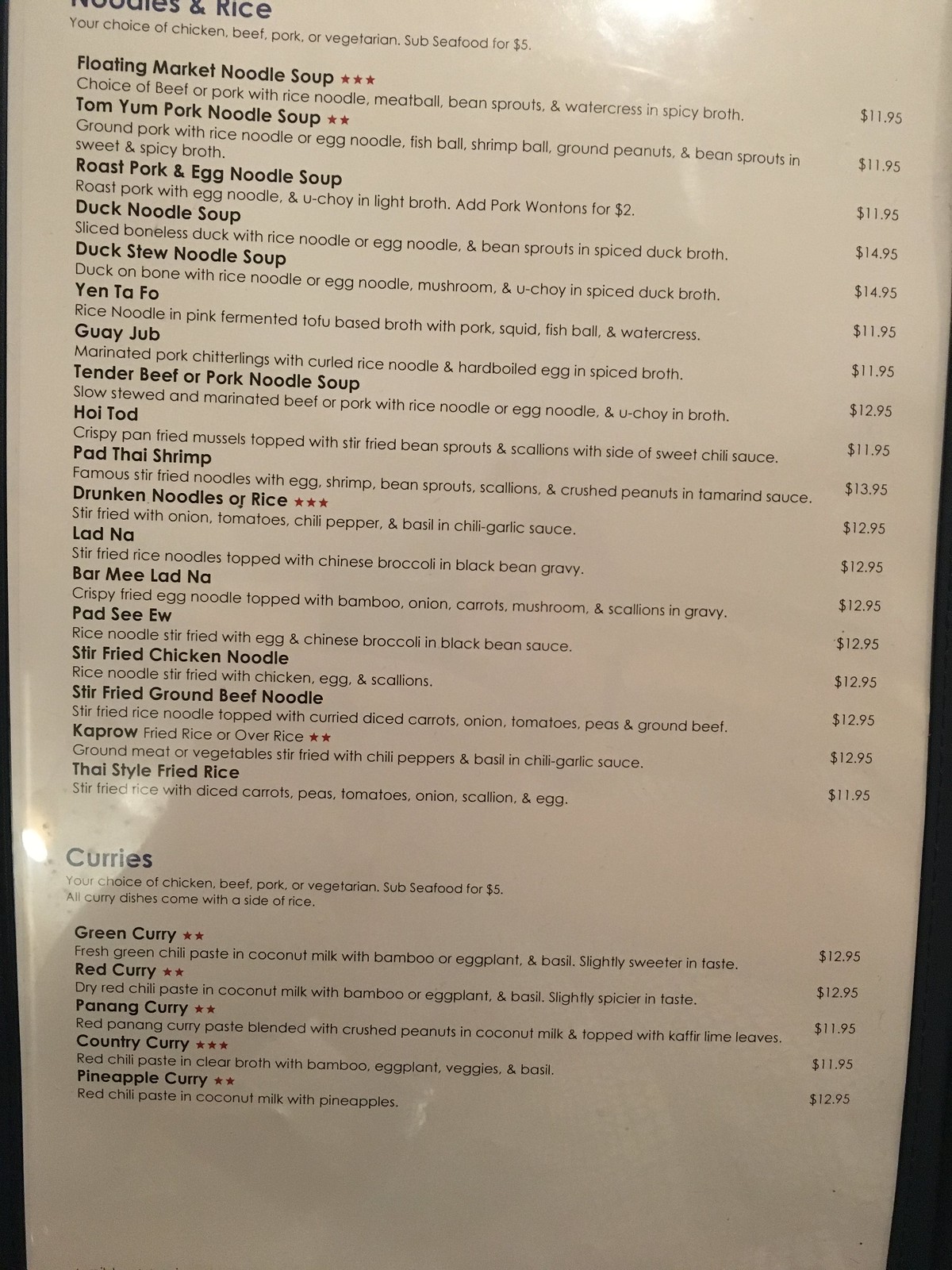The image captures a laminated menu, likely from a restaurant, characterized by its glossy surface which reflects the overhead lighting, creating a pronounced white glare at the top and along the side. The visible content begins with a section titled "Noodles and Rice," which offers a choice of chicken, beef, pork, or vegetarian options, with an additional $5 charge for substituting seafood. This section includes a variety of soups and rice-based dishes, with prices ranging between $11.95 and $14.95.

Below this, there is a section labeled "Curries," which similarly presents options of chicken, beef, pork, or vegetarian, and allows seafood substitution for an extra $5. Each curry dish is accompanied by a side of rice. The prices in this category span from $11.95 to $12.95. The menu is set against a black background, though the image capture is incomplete, cutting off the top portion including part of the titles "noodles" and "rice," trimming through the "R" and part of the "I" in "rice."